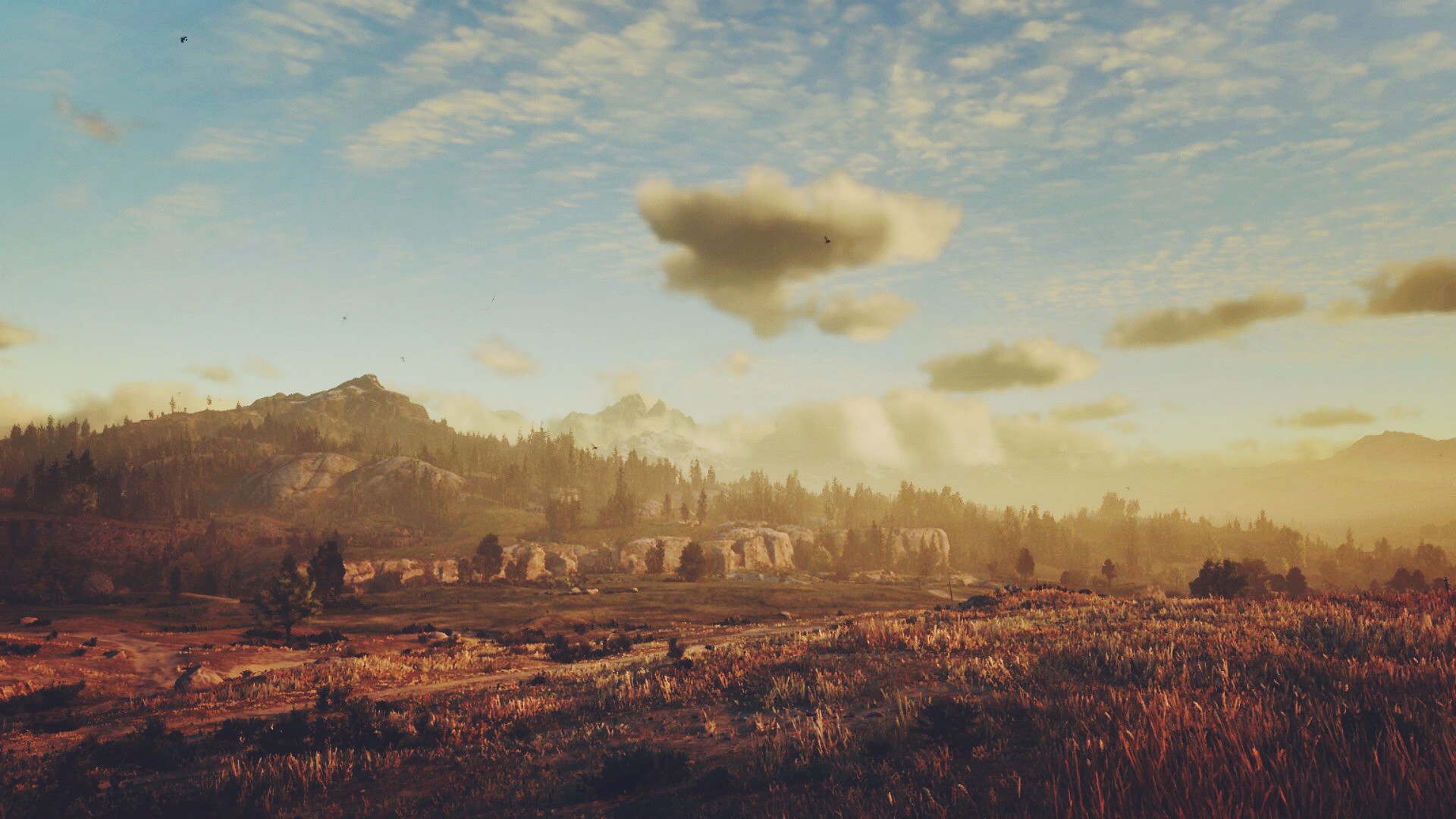The image appears to be a detailed painting of a sprawling landscape, primarily featuring a large horizontal swath of reddish-brown land. This terrain is dotted with short brush or plant life. Moving into the midground, the expanse transitions into rocky cliffs and foothills adorned with tall, dense evergreen trees. Interspersed among the vegetation, there seems to be a series of stone houses or a small hamlet, which adds a human element to the natural scene.

In the background, the rocky hills rise up, leading to densely packed forests that cover the slopes. Beyond these hills, more rugged mountains loom, partially shrouded by a mix of wispy and dense white clouds. The sky above these mountains is a vivid light blue, though it is partially obscured by these clouds. Notably, there are a few larger, darker clouds positioned closer to the viewer, suggesting an impending change in weather.

In the foreground, the ground is characterized by a mix of brown grass and scattered rocks, giving it an earthy, textured appearance. The entire scene is suffused with a slight haze, particularly towards the background, lending a sense of depth and atmospheric perspective to the painting.